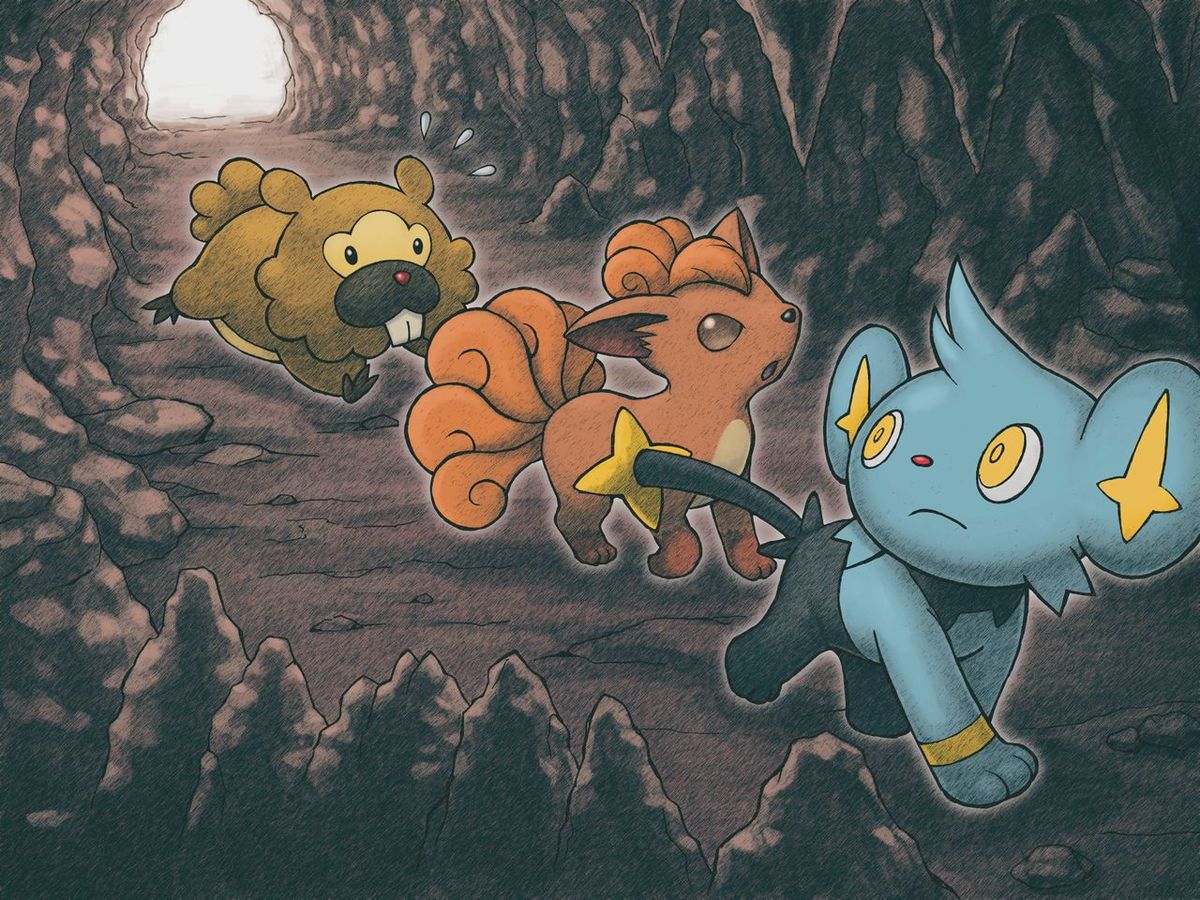In this cartoon drawing, three unique and colorful animals are depicted moving through a dimly lit cave. The entrance of the cave, a gray opening, is positioned in the upper left section of the image, hinting at the transition from the outside world into this cavernous environment. The walls of the cave are illustrated using a palette of dark browns and tans, which progressively darken as the cave extends deeper into its depths.

Leading the trio is a blue, cat-like creature that is moving on all fours. This character has rounded ears, adding to its distinctive feline appearance, and appears to be male. The blue creature is dressed in black pants that extend all the way to its tail, which is decorated with a yellow star shape at the tip.

Following closely behind is another cat-like animal, but this one has a tan and reddish-brown coat. The creature boasts a very fluffy tail and features stylized, puffy hair nestled between its pointy ears, suggesting it is female.

The final member of the group is a beaver-like creature, characterized by its brown and tan coloration. This animal has a distinctive black area around its red nose and two pronounced front buck teeth. It adds to the diverse and lively ensemble navigating the cave's interior.